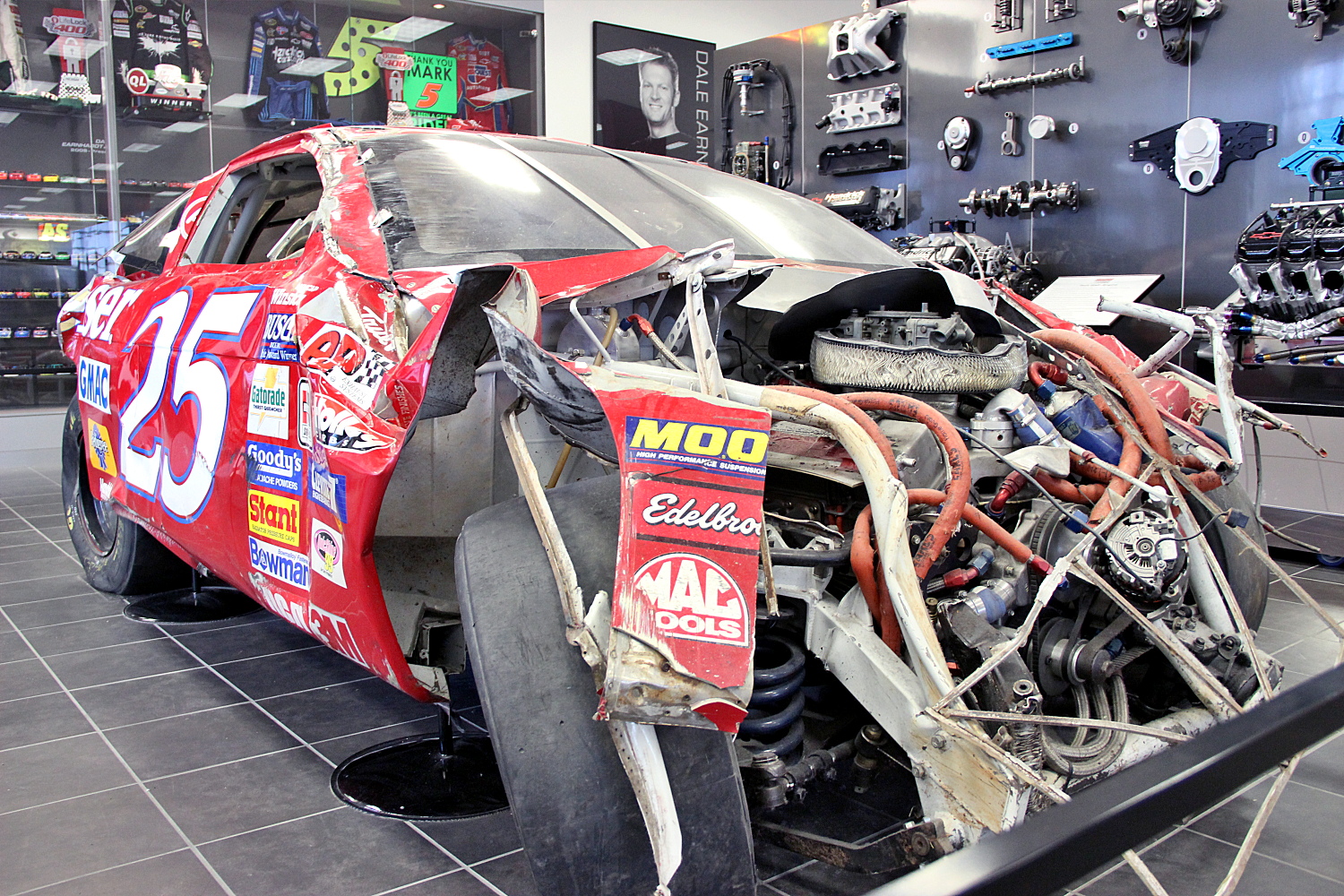In this detailed image, we see a highly damaged red race car prominently displaying the number 25. The car appears to be in a museum or a private collection room, dedicated to racing memorabilia. The front end of the vehicle is severely smashed, with the hood and fenders completely missing, exposing the inner workings and the engine. The vehicle is elevated on jacks, suggesting it's held up for display or inspection. The wheels are bent, and one of the back tires shows significant denting. The floor beneath the car displays stains, possibly from oil or other fluids dripping from the damaged frame. Surrounding the wrecked car, the setting features a gray-tiled floor, a gray wall adorned with various car parts, engines, and tools. Behind the car is a glass display case containing uniforms, plaques, and other racing paraphernalia, including a Dale Earnhardt poster, which reinforces the museum-like atmosphere.